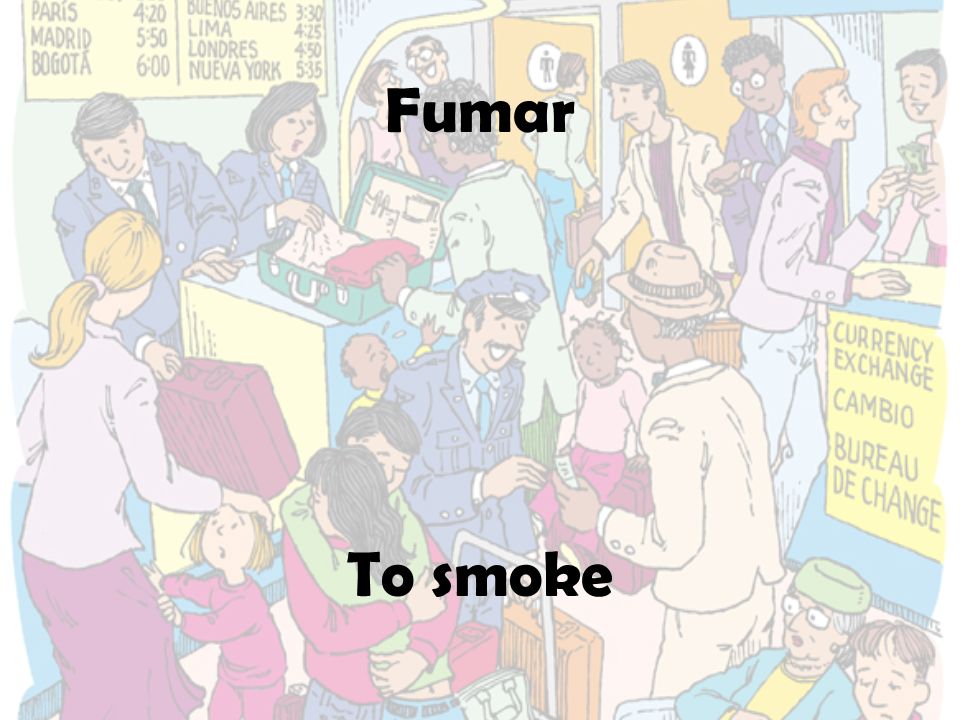The image presents a busy, cartoon-styled airport scene with vibrant colors like red, pink, blue, yellow, black, brown, and white. The central focus is on a multitude of people engaged in various airport activities. In the upper middle part of the image, bold text reads "FUMAR" with the translation "to smoke" below it. A flight announcement board on the upper left side lists destinations and times: Paris 420, Madrid 550, Bogota 6, Buenos Aires 330, Lima 425, Londres 450, and Nueva York 535, all in black letters on a yellow background.

The right side displays a currency exchange booth marked with "currency change," "cambio," and "bureau de change." Numerous characters populate the scene, including men in blue uniforms with white shirts and ties, some wearing blue hats with badges, and individuals in pink outfits. There are people sitting and waiting, others greeting each other, and security personnel inspecting baggage with an x-ray machine. The upper area includes male and female bathroom doors with stick figures indicating gender. The overall feeling is one of lively activity, typical of an international airport terminal depicted in an artistic and somewhat blurry cartoon rendering.